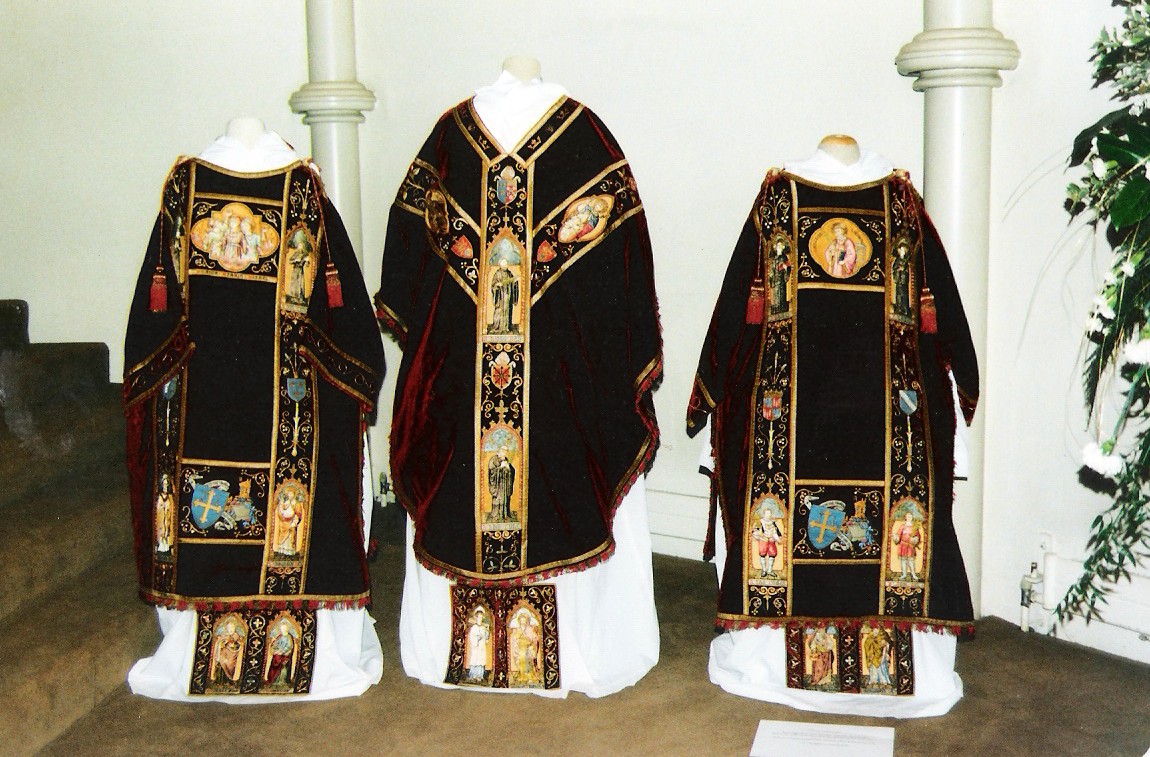The image depicts three intricately designed black robes, each adorned with elaborate gold detailing and abstract artwork, displayed on headless mannequins against a white background. The robes, possibly fashioned from velvet or corduroy, each exhibit unique patterns imbued with religious motifs, including crucifixes and figures. The designs suggest that these garments could be ceremonial attire for priests or regal gowns for royalty. The room, featuring white walls, two small pillars, and a brown carpeted staircase, enhances the regal and sacred ambiance. To the right, a green leafy plant adds a touch of organic contrast to the scene.